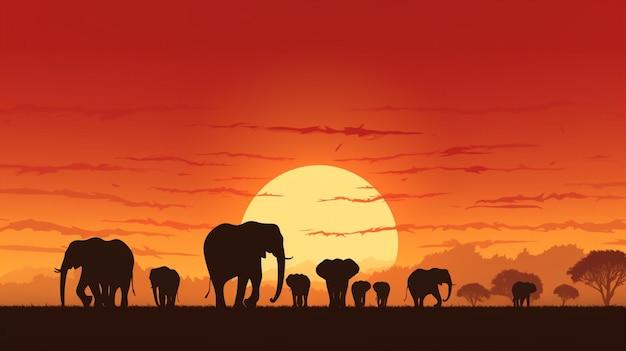In this stunning image, likely depicting the African plains, we are greeted by a breathtaking sunset. The sky transitions beautifully from vibrant dark red at the top, through lighter red, to a warm orange near the horizon, blending with the golden hues of the setting sun. Wisps of clouds meander through the sky, adding a delicate texture to the vivid colors. Dominating the image are the silhouettes of several elephants, both adults and smaller ones, standing majestically in the center. The backlighting from the sun renders the elephants in striking black silhouettes, their shapes impeccably clean and distinct, almost cartoonish in their precision. The terrain below them is a featureless, flat grassland, also captured in deep silhouette. Sparse trees are scattered throughout the scene, with a few closer to the foreground and many more dotting the distant horizon, their forms also absorbed into the dark outlines. The realistic yet artistically clean appearance of the elephants and the contrasting colors make it difficult to discern if the image is a real photograph or a digitally enhanced or painted scene, but its beauty and evocative atmosphere are undeniable.